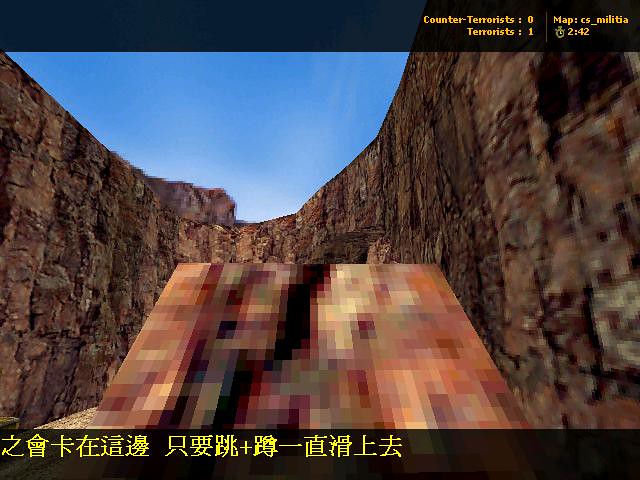The image appears to be a scene from a video game, featuring Asian characters at the bottom of the frame. On both the top and bottom borders, there are strips displaying various pieces of information. At the top, there is a scoreboard showing "Counter-Terrorists" and "Terrorists" with a score of zero to one, respectively. 

The central focus of the image is a colorful, slightly faded and blurry depiction of an environment resembling a canyon or a rocky area, with a map named "Militia" visible and a timer set at 2:42. The scene is composed of numerous intermingling boxes in various colors, adding to the abstract aesthetic. The viewpoint seems to be looking upward, framed by thick rock walls that encase the scene, and the sky above is a clear blue. The rocks are rendered in deep, earthy tones, providing a stark contrast to the vivid sky.